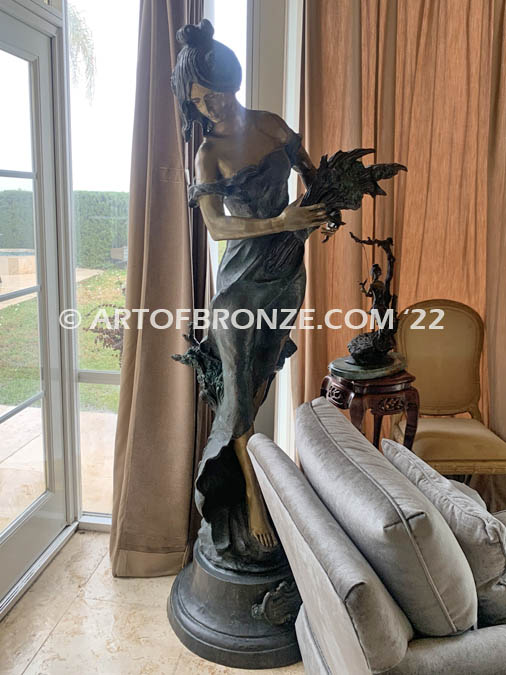The image displays an amateurish vertical rectangular photograph of a bronze statue located in a cluttered living room. The central focus is on a beautifully sculpted statue of a young woman with her hair styled in a bun, adorned in a flowing, off-the-shoulder gown that features a high slit and she's barefoot. She is elegantly poised, standing straight yet leaning slightly to one side, her head tilted downward as she tenderly cradles a bouquet of flowers. The statue, resting on a black base, is artistically captivating but poorly composed within the frame, partly obscured by an armchair that blocks the lower portion. A smaller bronze statue is placed on a table to the statue's right. The room itself is characterized by mismatched furniture and a window with open curtains revealing an overcast, muggy day outside. The image bears a watermark reading "artofbronze.com," copyright 2022, centered at the bottom.